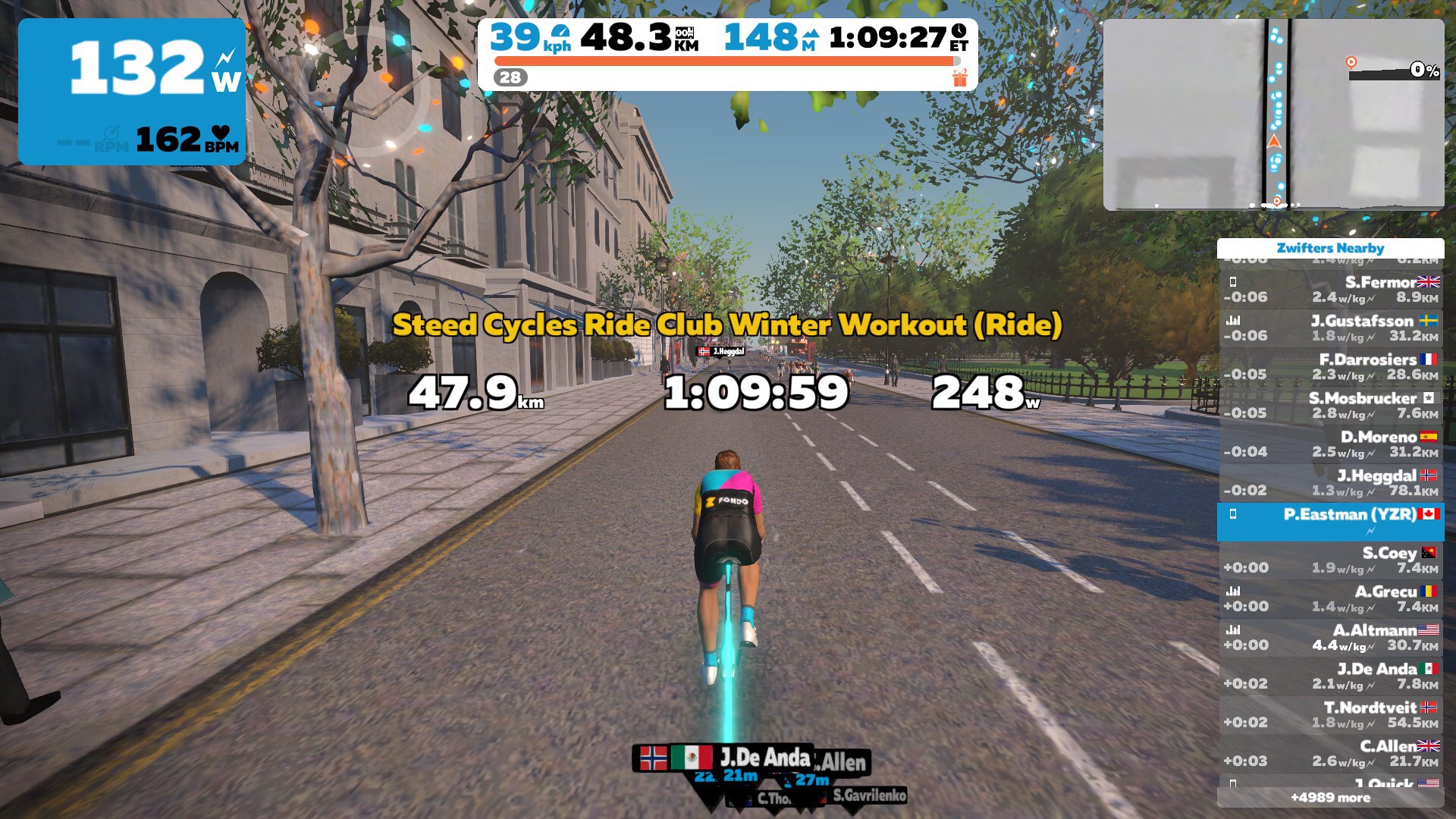The image is a detailed screenshot from a digital bicycle racing video game. At the bottom center, a cyclist dressed in black shorts with a blue and pink top and a brown helmet rides a bicycle with glowing blue wheels. The cyclist is on a gray road bordered by sidewalks with trees on either side, and a large building on the left.

The top of the screen displays various game metrics: a white horizontal bar shows the cyclist's speed at 39 kph, their total distance covered at 48.3 km, and their elevation at 148 meters. A detailed time tracker reads 1 hour, 9 minutes, and 27 seconds (ET). The upper-left corner features a blue box displaying power output at 132 watts and a heart rate of 162 BPM. 

The top right corner contains a mini-map outlining the race course, alongside a list of competitors' names and their placements, showing S. Ferner in first place and J. Gustafson following. The background image sets the scene with a gray road, double yellow lines on the left, white center markings, a parked car, trees, and urban scenery. 

At the bottom center, in yellow text, it reads "Steed Cycles Ride Club Winter Workout (ride)" followed by "47.9 km" and a time duration of "1:09:59" along with power output "248W" in white text. Flags and names of other participants, such as Pete Eastman, YZR, and their national flags appear, illustrating active competition. The immersive environment of the game provides a vibrant and dynamic cycling experience.